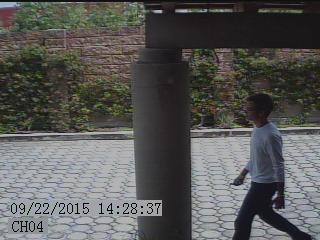This image is a still from an outdoor surveillance or security camera, captured on September 22, 2015, at 2:28:37 PM, labeled as CH-04. The scene showcases a man with dark hair, wearing glasses, and dressed in a white long-sleeve shirt and dark pants, possibly dark sneakers. He is walking from the right to the left side of the frame, along a wide cobblestone street or sidewalk, which features a metal pillar in the foreground. The man appears to be holding car keys in his right hand. In the background, there is a brick wall adorned with greenery, suggesting vegetation growing on it.